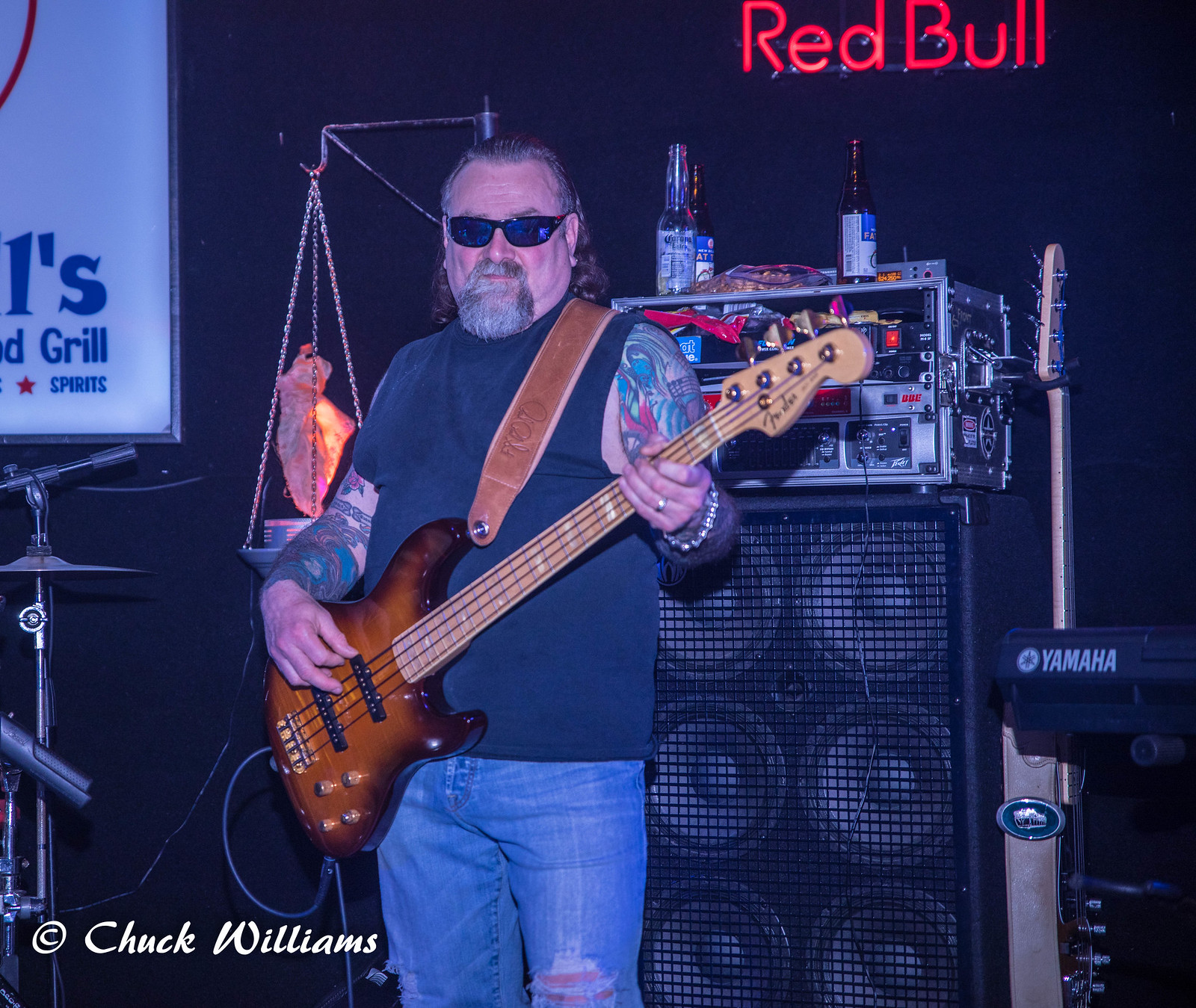The image depicts an older white gentleman, identified as Chuck Williams by the white text stating his name in the lower left-hand corner. Chuck is standing slightly to the left of the image, playing an electric bass guitar, which is brown and has four strings with a strap over his shoulders. He has long, slicked-back gray hair, a gray goatee, and is wearing sunglasses. His arms, covered in tattoo sleeves, are visible as he's dressed in a black cut-off t-shirt. He also has on ripped blue jeans, revealing a tear in the left knee. A wedding ring is visible on his finger.

The setting appears to be indoors, featuring several musical instruments and equipment. Directly behind Chuck are large speakers with beer bottles on top, an upright guitar, and to his left, a drum set. There is also a Yamaha keyboard positioned to the right side. The background includes a Red Bull neon sign and another indistinguishable silver object atop the speaker. The scene gives off a casual, yet intense musical vibe, possibly at a bar or a small venue, evoking a rock or blues atmosphere.